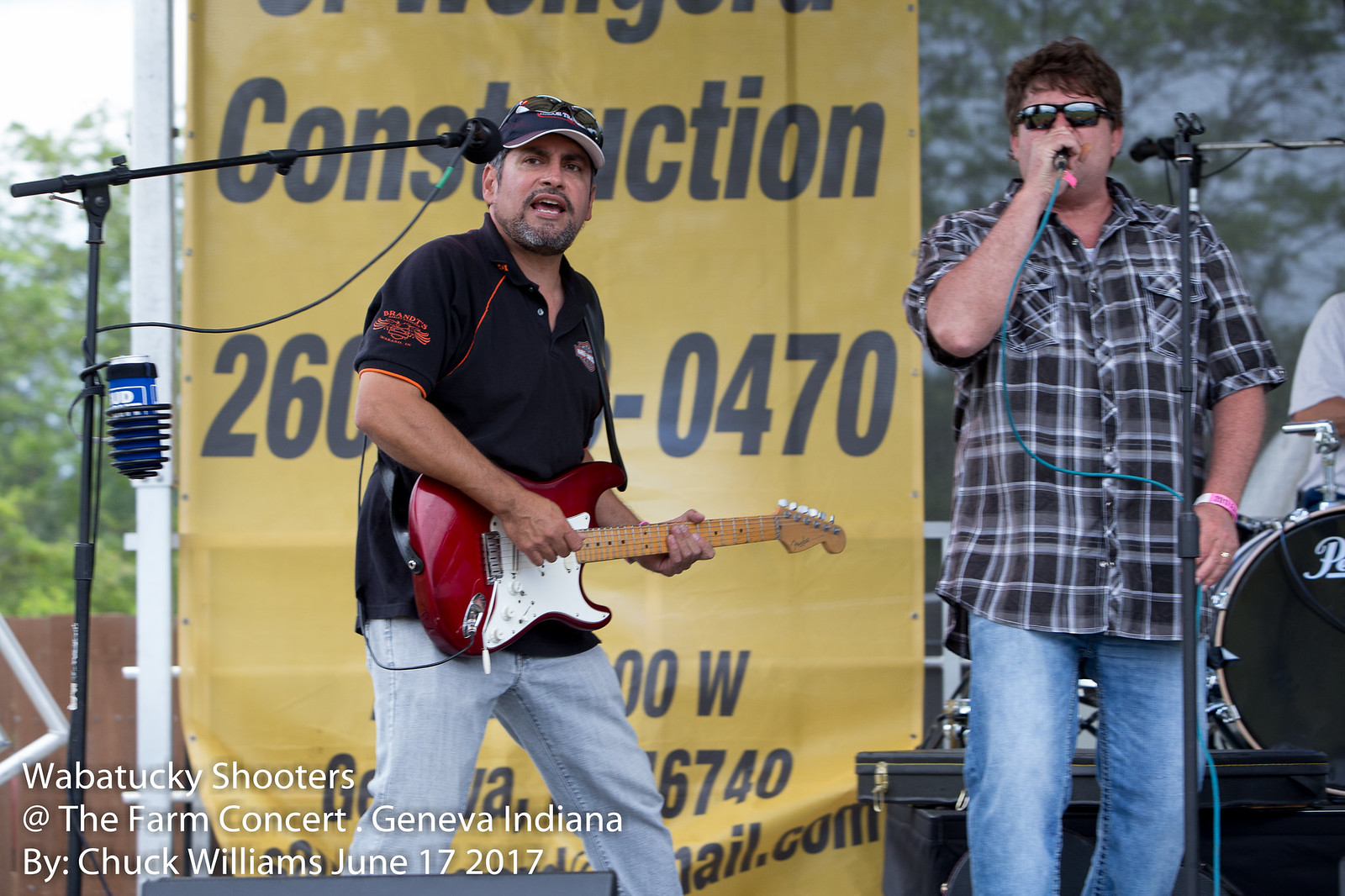The image captures a vibrant outdoor concert scene featuring three musicians on stage. At the center, slightly towards the left, stands a man wearing a black short-sleeved shirt with designs, a black cap, and sunglasses perched on the cap. He has a goatee and speckled gray hair, and is playing a red and white electric guitar. A black microphone is positioned at his mouth, and he has a blue koozie holding a Bud Light can attached to his mic stand. This guitarist is also in light-colored blue jeans and stands looking out at the crowd. To his right, another performer sings into a microphone, dressed in a grayish flannel shirt, blue jeans, dark sunglasses, and a pink wristband on his left wrist. Behind them, partially visible, is the drummer, wearing a white T-shirt, seated at a black and white drum kit. The backdrop features a large yellow banner with the word "construction" and partially obscured contact details. Adding context to the scene, the bottom left corner of the image displays text: "Wabatake Shooters at the Farm Concert, Geneva, Indiana, by Chuck Williams, June 17, 2017." The setting is outdoors amidst trees, under a bright daytime sky, creating a lively and engaging atmosphere.